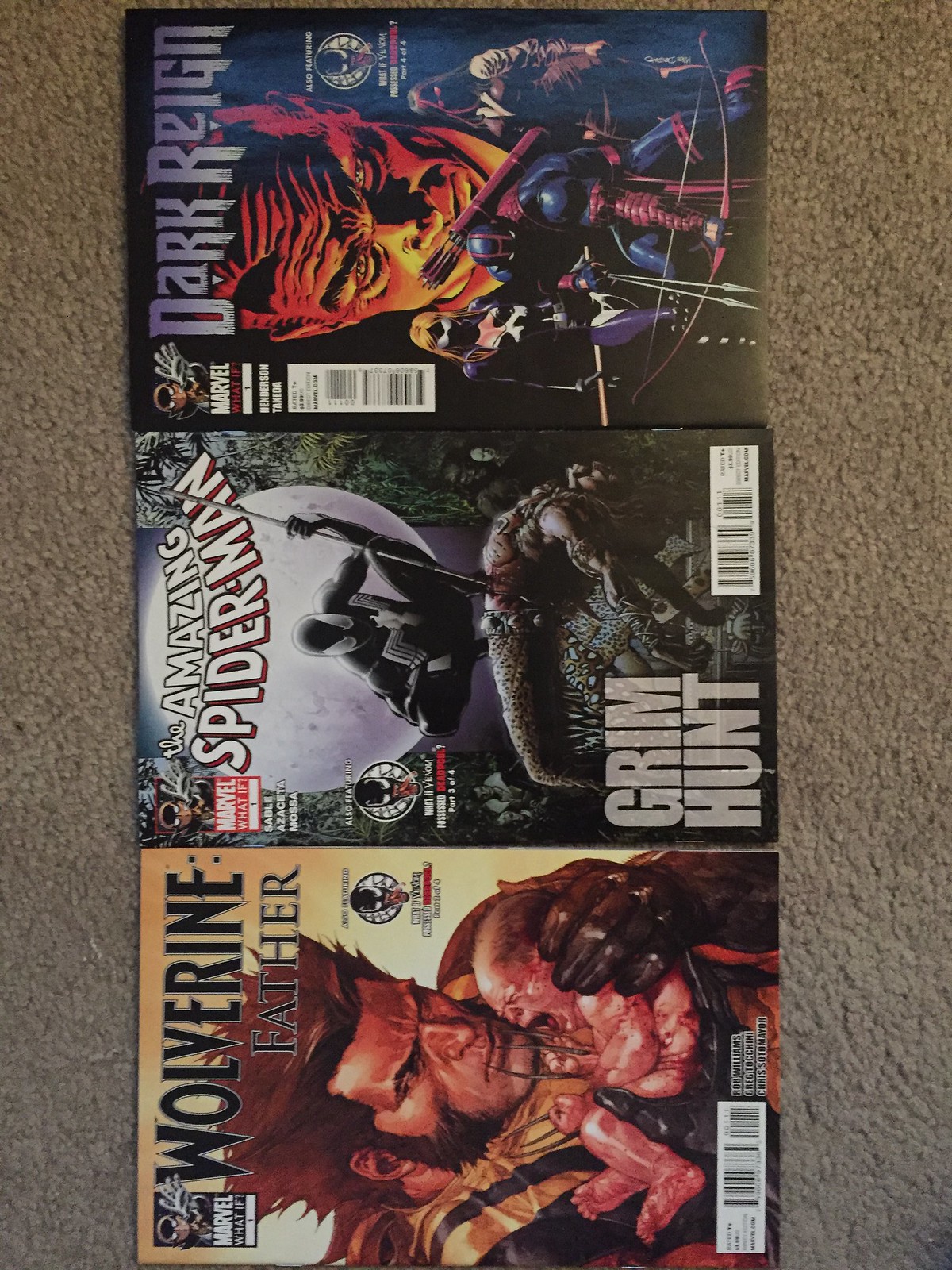The image captures three comic books arranged horizontally on an outdoor asphalt surface, photographed at an angle that makes them appear vertical. The first comic on the left, titled "Wolverine Father," features Wolverine holding a baby, with the words "Marvel What If" in the top left corner. The middle comic, "Amazing Spider-Man: Grim Hunt," depicts Spider-Man as he appears to impale an arched figure with a spiky pole, set against a backdrop of the moon and eerie, white-faced characters. The last comic, "Dark Reign," showcases a face bathed in red, green, and yellow tones, surrounded by maskless figures, including women gazing downward and a man with bow and arrows on his back. Each comic features a barcode, confirming their identities as publications rather than DVDs or games.